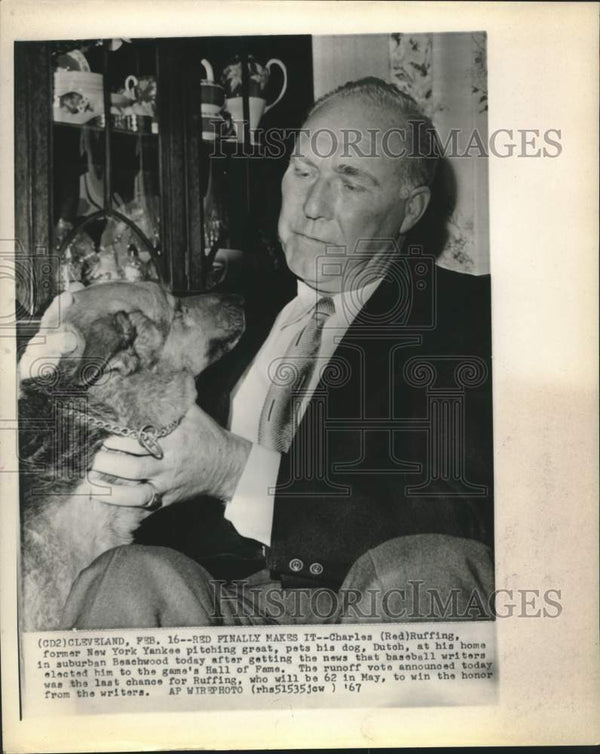This is a vintage black-and-white photograph featured on aged white paper, likely from a book or newspaper clipping, with watermarks stating "Historic Images" at the top and bottom. A large watermark in the center depicts a camera on a pedestal. The photo shows an older, partially balding man seated and wearing a suit—dark blazer, white collared shirt, gray slacks, and a light-colored tie. This man, identified as Charles "Red" Ruffing, a former New York Yankees pitching great, is affectionately holding and petting his large dog Dutch, which resembles a German Shepherd and wears a choke chain collar. Below the image, text reads: "CD to Cleveland, February 16th. Red finally makes it. Charles 'Red' Ruffing, former New York Yankee pitching great, pets his dog Dutch at his home in suburban Beachwood today after getting the news that baseball writers elected him to the Games Hall of Fame. The runoff vote announced today was the last chance for Ruffing, who will be 62 in May, to win the honor from the writers." Additional text notes, "AP wire photo (RHA 5 1 5 3 5 JC W '67)."